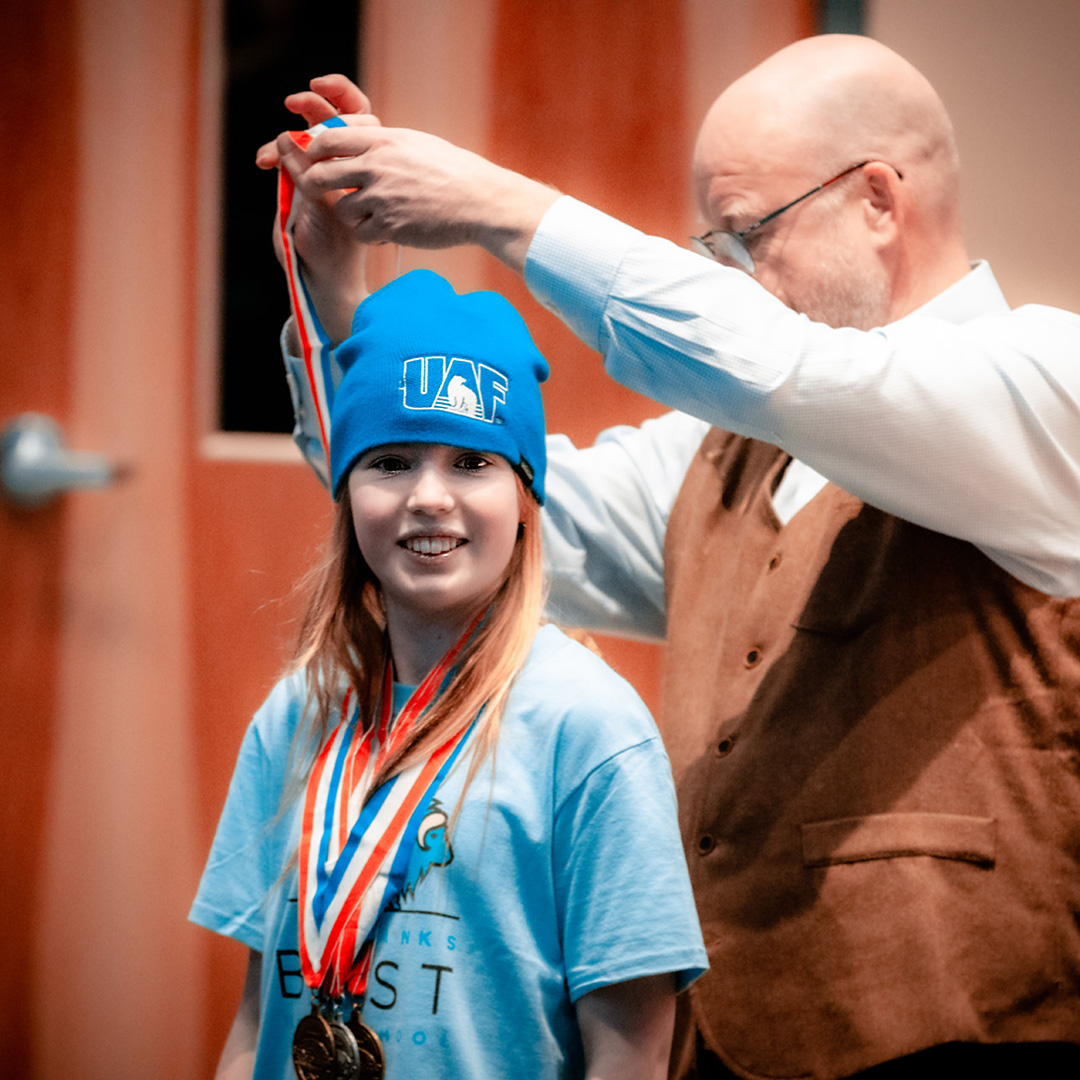The photograph captures an elderly white man with glasses and a brown vest over a long-sleeved white shirt, as he places a medal around the neck of a young girl. The young girl, who has chest-length red hair, is facing the camera and smiling, showcasing her big front teeth. She is wearing a blue beanie adorned with the initials "UAF" and a polar bear on the letter A, as well as a light blue T-shirt with the word "best" visible. The girl already has three medals on red, white, and blue ribbons around her neck: two bronze and one silver. They appear to be in an auditorium, with a distinctive orangey wood-colored door with lighter stripes and a silver industrial handle in the background. The scene captures a moment of joy and accomplishment as the man awards another medal to the beaming girl.